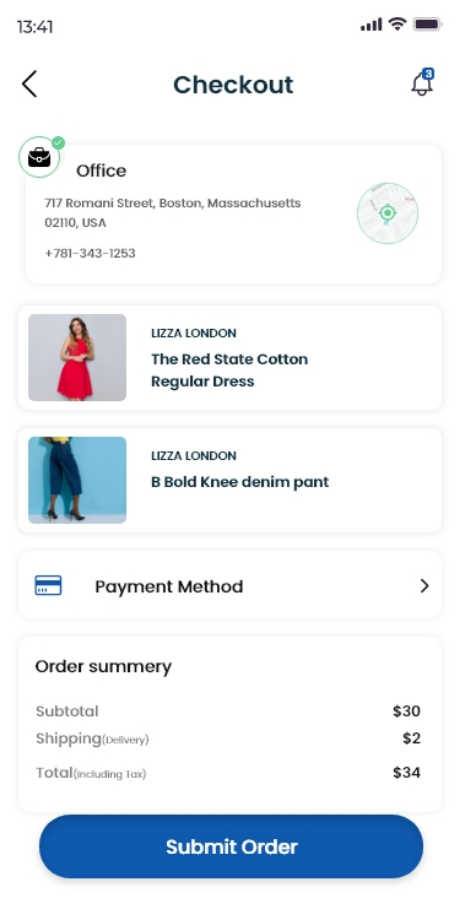A detailed screenshot of a smartphone shows a white background with the time displayed as 13:41 in black at the top left corner. In the upper right-hand corner, there are four bars representing the Wi-Fi signal and a fully charged black battery icon. Below, in large black letters, the text reads "Check Out," with a notification bell to the right that has a green bubble with the number "3."

The screen is divided into three sections related to the checkout process. In the upper left corner of the first section, there's a briefcase icon followed by a green circle containing a white check mark. To the right, the word "Office" is displayed in black, along with an address and phone number.

The second section lists the purchased products. On the left, there's an image of a young woman with long blonde hair wearing a red dress, labeled "Liz of London." The description indicates the purchase of a "Red State Cotton Regular Dress." Another item displayed on the left, set against a blue background, shows black capri pants labeled "Liz of London: Be Bold Knee Denim Pant."

Below this, a credit card icon on the left is followed by the text "Payment Method," with a right-arrow icon on the right.

The final section, titled "Order Summary," details the costs: subtotal $30, shipping $2, and a total of $34. At the bottom, there is a rectangular dark blue button with "Submit Order" written in white lettering.